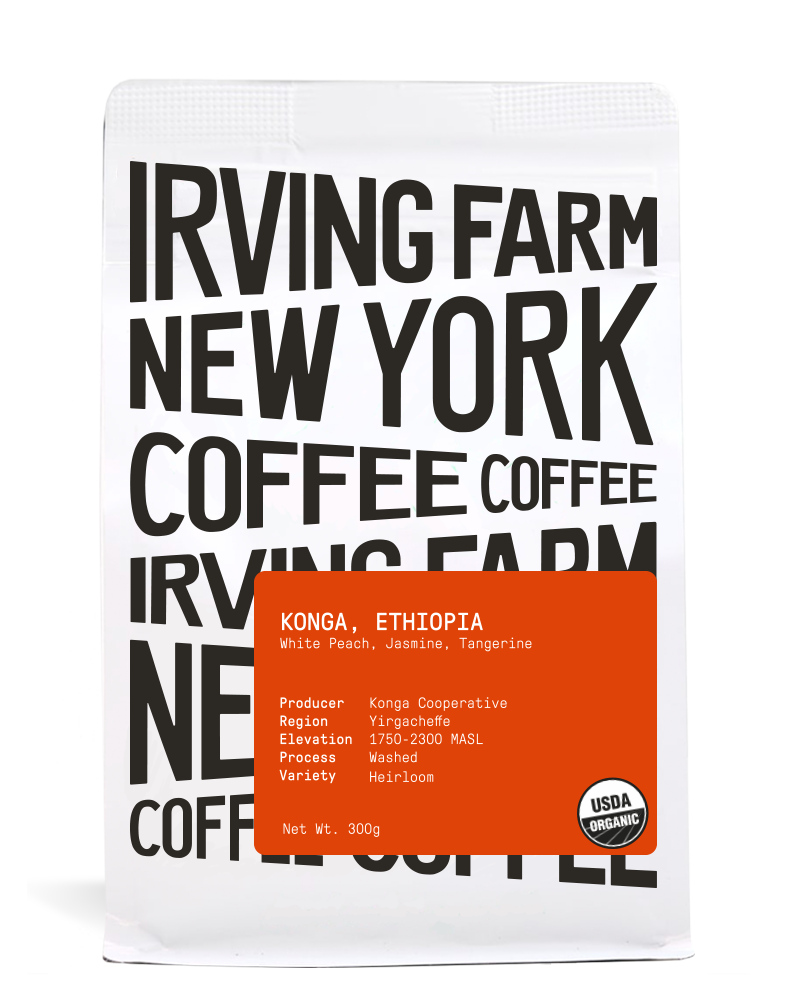The image is a detailed close-up of a pouch of coffee with a white foil bag. The design prominently features a series of large black letters in varying angles and sizes repeating "Irving Farm New York Coffee" across the front of the bag. An orange square is situated in the lower right corner of the bag, containing white text that details the coffee's origin: "Conga, Ethiopia," along with tasting notes of "White Peach, Jasmine, and Tangerine." This square also provides information about the producer, region, elevation, process, and variety of the coffee. Additionally, a black and white USDA organic logo is located at the bottom right corner, emphasizing the organic quality of the coffee. The net weight is listed in the bottom left corner of the label. The overall design is reminiscent of an 8x11 poster with a white background and varying black block letters, presenting a visually striking and informative package.